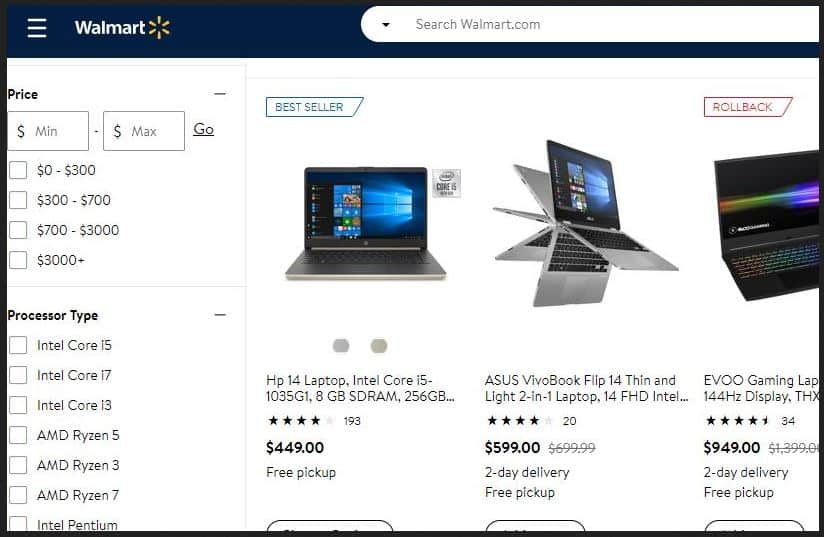This image captures a screenshot of the Walmart app interface. The app features a prominent blue navigation bar at the top, which spans the width of the screen. In the upper left corner, there's a three-horizontal-bar icon indicating a menu. To the right of this icon, the Walmart brand name is displayed in white, accompanied by the store's iconic yellow spark logo. Further to the right, there's a search bar with a dropdown arrow at the far end, facilitating easy searches.

Below the navigation bar, there's a price range filter section with two input boxes for minimum and maximum prices, and a "Go" button for applying the selected range. Under this, there are four checkboxes for different price ranges: "$0 to $300," "$300 to $700," "$700 to $3,000," and "$3,000+," all of which are currently unchecked.

Further down, there’s a section labeled "Processor Type" in black text. This section includes several unchecked boxes listed vertically, each associated with various processor options: Intel Core i5, Intel Core i7, Intel Core i3, AMD Ryzen 5, AMD Ryzen 3, AMD Ryzen 7, and Intel Pentium.

On the right side of the page, there is a visual display of laptops. Three laptops are displayed horizontally in a row. Above the first laptop on the left, there's a "Bestseller" tag, and above the third laptop on the right, there's a "Rollback" tag, indicating special promotions.

The detailed layout and clear labeling make it easy for users to navigate through different product filters and view featured laptops.